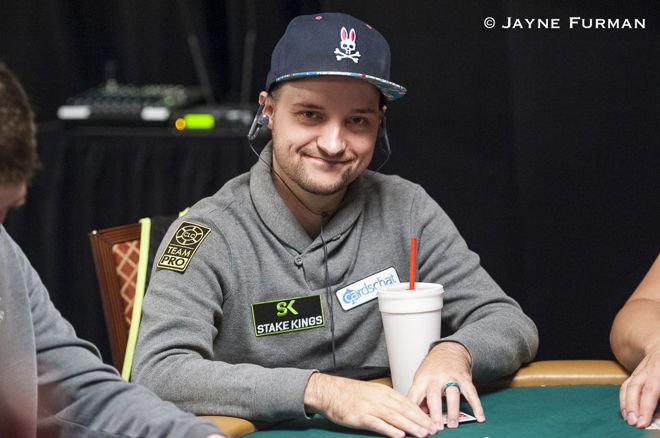In this detailed freeze-frame from a live poker tournament, captured by Jane Furman, a Caucasian man is the central focus. He sports a black baseball cap featuring a skull and crossbones with bunny ears and a plaid brim. Wearing a gray pullover adorned with several patches—'Team Pro,' 'Steak Kings,' and 'Cards Chat'—the man appears deeply engaged in the game. With a slight smile and a faint beard, he looks directly at the camera, his teeth not showing.

The poker player's left hand, adorned with a wedding ring, hides the backs of red cards that rest on the green felt table. A headset is attached to his ears, suggesting he might be communicating or listening to something pertinent to the game. In front of him sits a white Styrofoam cup with a red straw, along with another drink nearby. The blurred background hints at a busy tournament setting with at least two other unidentified participants partially visible. The overall atmosphere exudes a professional and focused intensity.